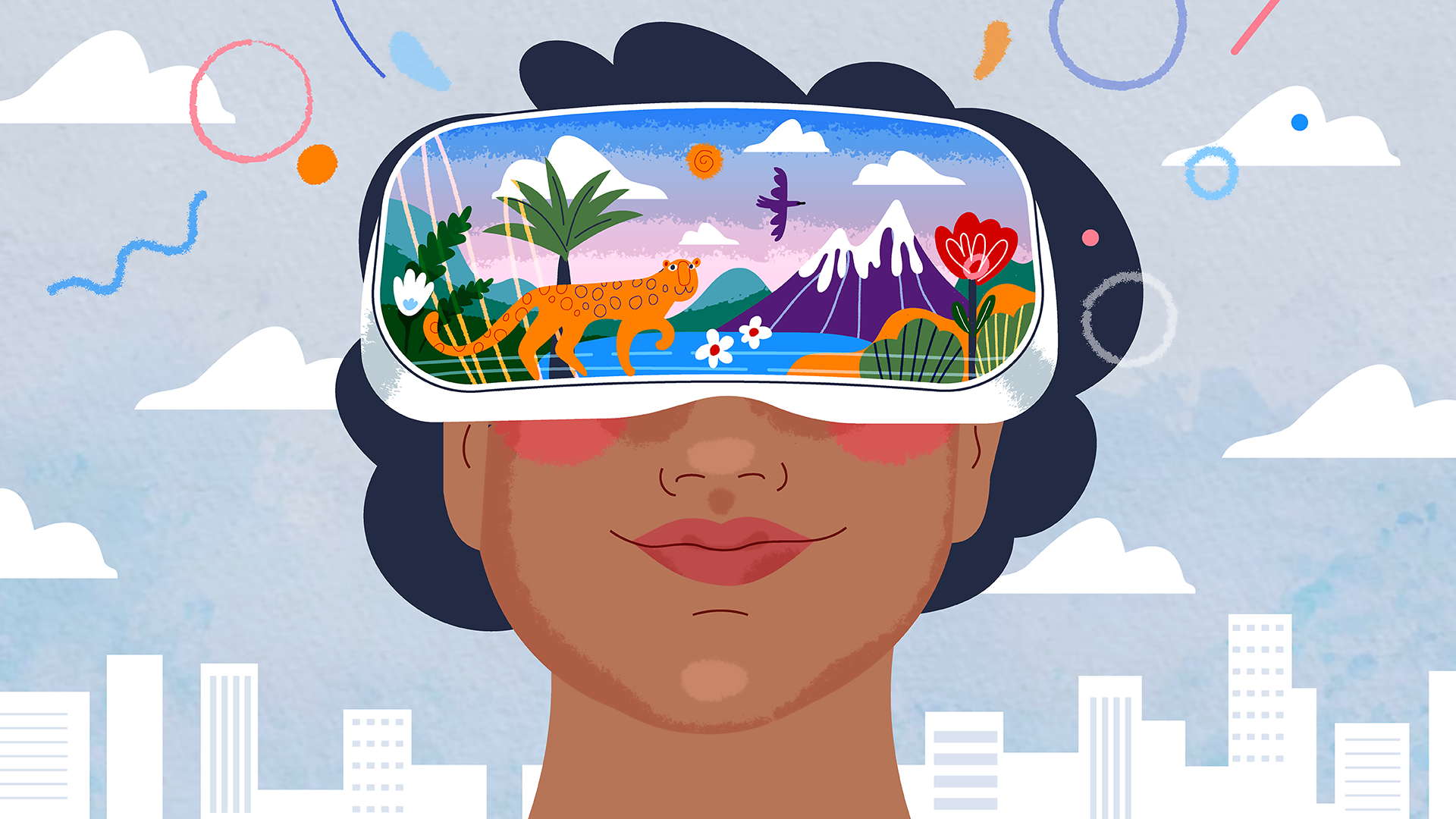The image is a digitally drawn cartoon of a smiling woman with dark brown skin and short, curly black hair, prominently centered. She is wearing a VR headset that completely covers her eyes. The headset displays a vivid nature scene featuring an orange and spotted big cat, possibly a tiger or cheetah, walking towards snow-capped mountains. The scene also includes a palm tree, green shrubbery, white and red flowers, a bird in flight, and a lake, all set against a sky of blues, purples, and pinks. The background of the full image shows a light blue cityscape with white clouds and simple, colorful doodles like squiggles and circles in orange, blue, pink, and red. The woman’s cheeks are slightly blushed, and her lips are a deep red. The main focus remains the woman with the VR headset, emphasizing the contrast between the digital urban backdrop and the immersive natural scene displayed in the headset.